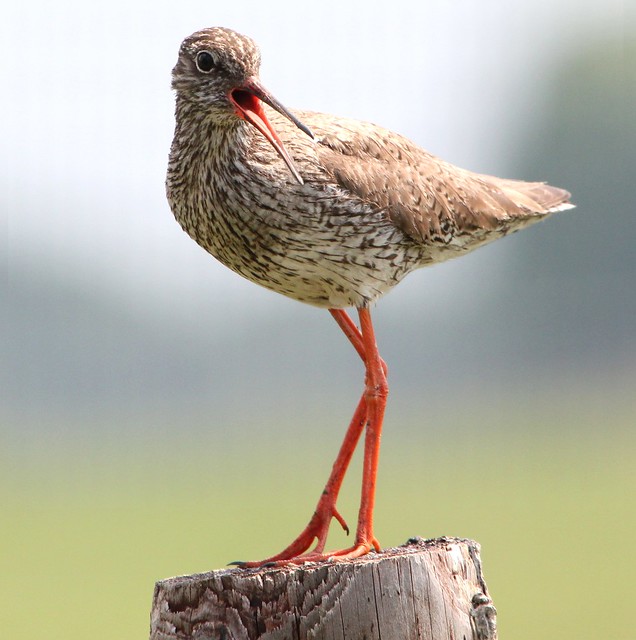The image is a close-up photograph of a bird standing on top of an aged, rotting gray tree stump, which is rich in broken-down texture. The bird is equipped with very long, thin, orange legs that culminate in small talons with noticeable black nails. This bird, relatively small in body size compared to its legs, displays a complex feather pattern of white, light gray, and dark gray, with specks and stripes of brown along its body. Its wings, a lighter shade of brown or off-white, are folded tightly against its sides. The bird has a longish neck and a small head characterized by a distinctly long, pointy beak, which is dark brown or black on the outside and orange on the inside. Its black eye stares intently at the camera, giving an impression of hunger or anger, with its beak open as if making a sound. The background, bathed in shades of gray and green, is heavily out of focus, ensuring that all attention is centered on the bird.